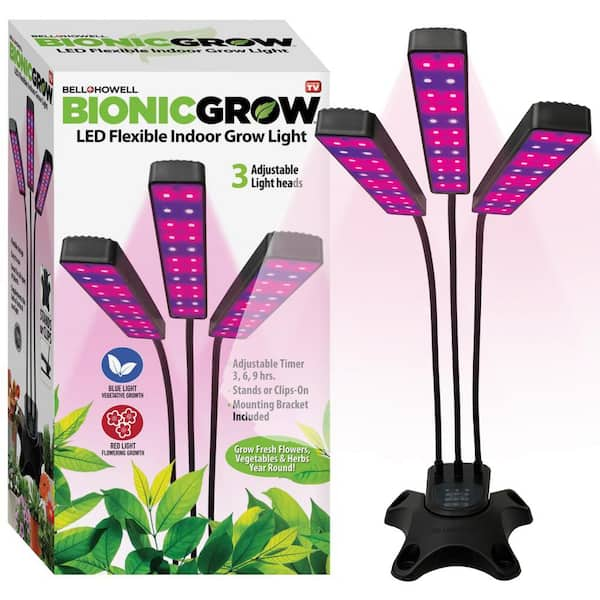The image is a detailed product advertisement for the Bell Howell Bionic Grow LED Flexible Indoor Grow Light. Dominating the right side of the image is the product itself, which consists of a sleek black base with three flexible poles, each culminating in an LED light panel emitting a combination of blue and red light, giving off a pinkish-purple hue. Each light head is attached to the pole, designed for optimal adjustment to target different plant areas. The assembly of the light heads and the flexible poles somewhat resembles a multi-head desk lamp. 

To the left of the product is the packaging, a pristine white box adorned with green plant leaves, contributing to a fresh and organic feel. The box prominently displays the product image and includes detailed information: Bell Howell Bionic Grow LED Flexible Indoor Grow Light, three adjustable light heads, an adjustable timer with settings for 3, 6, or 9 hours, and the flexibility to either stand independently or clip on, with a mounting bracket included. The well-known "As Seen On TV" logo adds a layer of credibility and familiarity at the top corner of the box. The box also highlights the intended use: growing fresh flowers, vegetables, and herbs year-round. The overall presentation is on a clean white background, enhancing the product's visibility and emphasis.